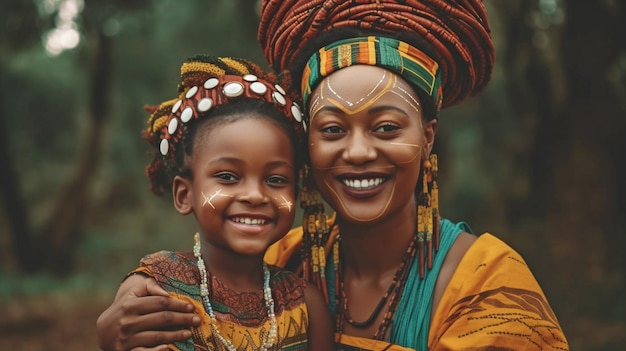In this vibrant photograph, an adult woman and a young girl, both with dark skin, are pictured amidst a lush background of green leafy trees. The woman, likely the girl's mother, has her arm affectionately wrapped around the child. Both are beaming with broad smiles; the girl gazing directly into the camera while the woman looks slightly to the right. 

They are adorned in traditional African attire, predominantly featuring colors like yellow, brown, and turquoise. The woman wears a headpiece adorned with red beads, combined with a yellow and white face makeup that outlines her features. Her accessories include long gold, brown, and aqua earrings, a matching necklace of brown beads, and a layered outfit comprising a teal cloth and a yellow dress or coat.

The girl, on the other hand, sports a white-disk headband and similar white makeup on her cheeks, accentuated by colorful beads. Their attire and adornments clearly reflect rich cultural heritage, possibly African or Jamaican, enhancing the warmth and joy captured in their smiles against the blurred, verdant backdrop.